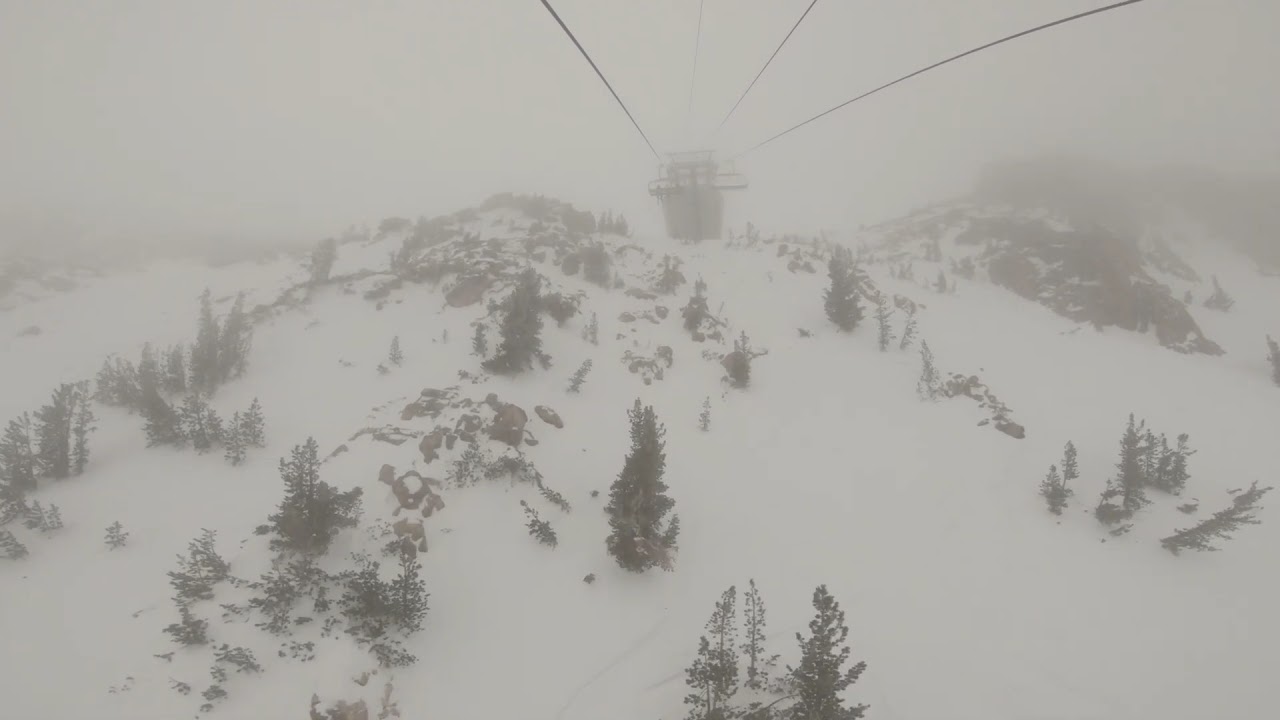The image is a photorealistic color photograph in landscape orientation, capturing a snowy landscape from the perspective of a raised gondola or chairlift. The scene presents a bird's-eye view of a large, snow-covered hill dotted with dark grayish coniferous trees, their colors muted by the lack of sunlight. Overhead, three thick cables stretch from the top right of the image into the foggy distance, suggesting they support the gondola or chairlift. In the bottom foreground, the ground far below is uniformly white with occasional dark green pine trees breaking through the snow. The landscape below is also marked by a rock outcropping on the top right side of the image.

In the middle distance, barely visible due to the enveloping white fog and overcast sky, lies what appears to be a building, likely a ski lift station where the cables converge. The sky is entirely white and gray, laden with fog or possibly falling snow, casting a hazy, dreamlike quality over the scene. The overall atmosphere conveys a cold and cloudy day, with the muted light filtering through the thick cloud cover. Another cable car is seen further along the cables, receding towards the distant building and adding depth to the vast, wintry landscape.